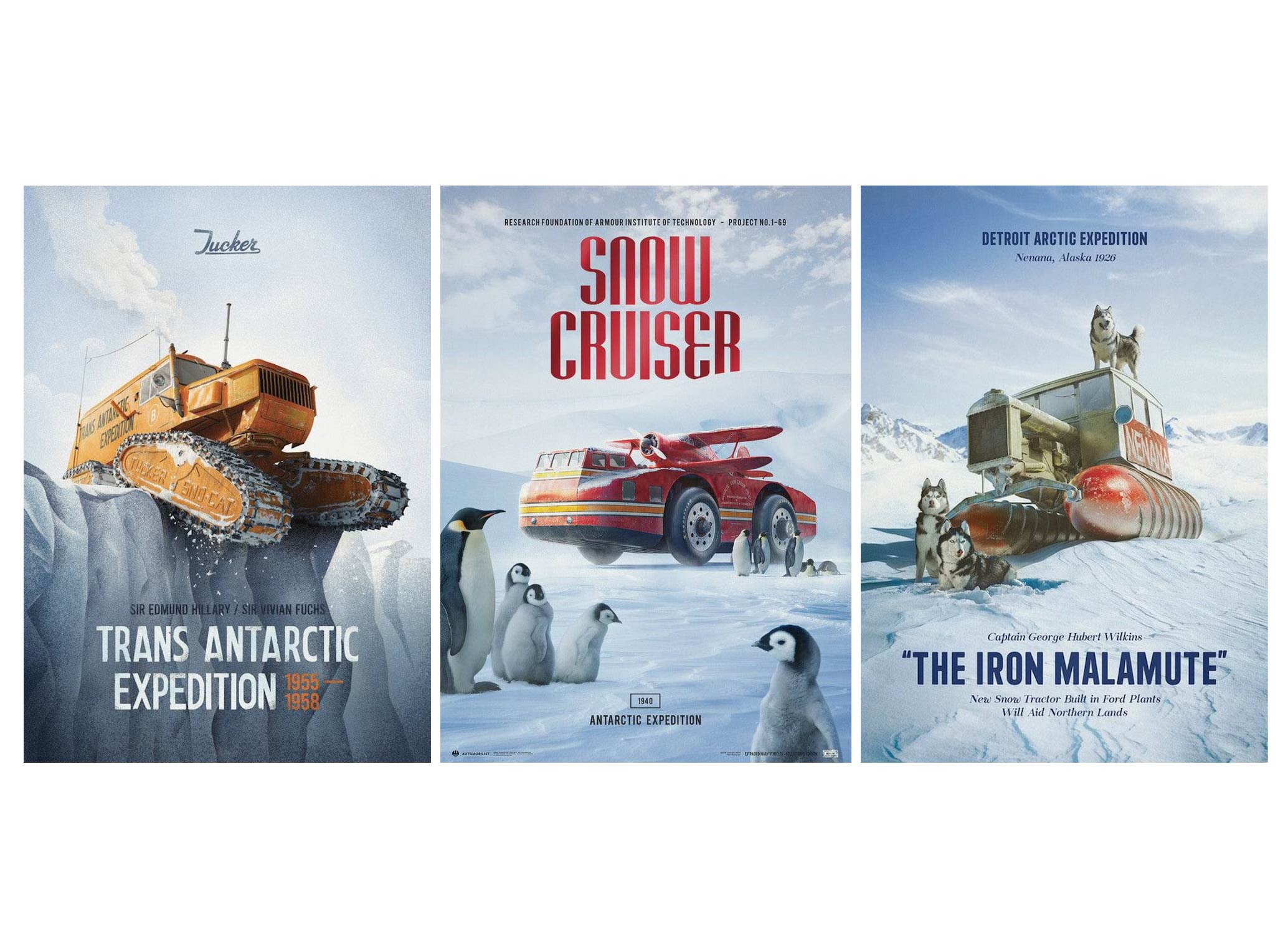The image features three distinct, snow-themed posters, each depicting a different scene from an Arctic or Antarctic expedition. 

The first poster, labeled "Transantarctic Expedition 1955-1958," shows a yellow tractor with a rectangular cabin and four sets of movable treads precariously hanging over the edge of an icy cliff. It has distinct aerial antennas and appears to be on a treacherous glacier edge under a cloudy, light blue sky.

The middle poster, titled "Snow Cruiser" in red, displays a red, hybrid vehicle with a cubic cabin and yellow-orange stripes. The vehicle is surrounded by various penguins, including emperor penguins with their young, against a backdrop of snowy or icy terrain, under a partly cloudy, blue sky.

The third poster, labeled "Iron Malamute," features a red, treaded vehicle with a rectangular cab on top, from which a Malamute dog is peering out. In front of the vehicle, there are two Malamutes on the snowy ground. The scene is set against a backdrop of distant icy mountains and a high, thin cloud cover in a blue sky. This poster also includes references to the Detroit Arctic Expedition and looks like an ad for an Arctic-themed film.